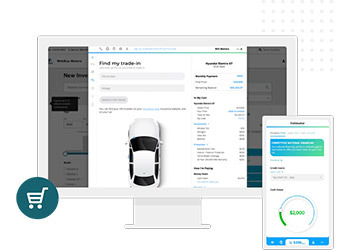This image features a white background with several distinct elements. In the bottom left corner, there is a dark blue circle containing a white shopping cart icon, with the handle oriented to the right. Dominating the central portion of the image is a sketched outline of a laptop. The laptop's screen depicts a website; its left and right sections appear slightly grayed out due to a central pop-up tab. This pop-up includes five icons aligned in the top left, blue lettering, and various pieces of information on the right.

Below the pop-up, the screen displays the phrase "Find My Trade-In" followed by three gray input tabs, with two extending more than halfway across the screen and the third about an inch wide. Additionally, there's a line of text underneath this section. The lower part of the laptop screen shows an image of a white car viewed from above its hood. To the right of this, there is some black, indistinct text, along with various details and price numbers aligned vertically.

The laptop itself has a grayish border. Above the device, there are four rows of dots arranged horizontally. On the right side of the laptop, another four rows of dots are aligned vertically.

Overlapping the laptop at the bottom, there is a depiction of a cell phone. The phone screen features a blue triangle containing some information and a dropdown tab situated about midway down. There's also a blue circle originating from the bottom left and arching up to the left center, then around to the right. Within this circle, the number "2000" is prominently displayed in green.